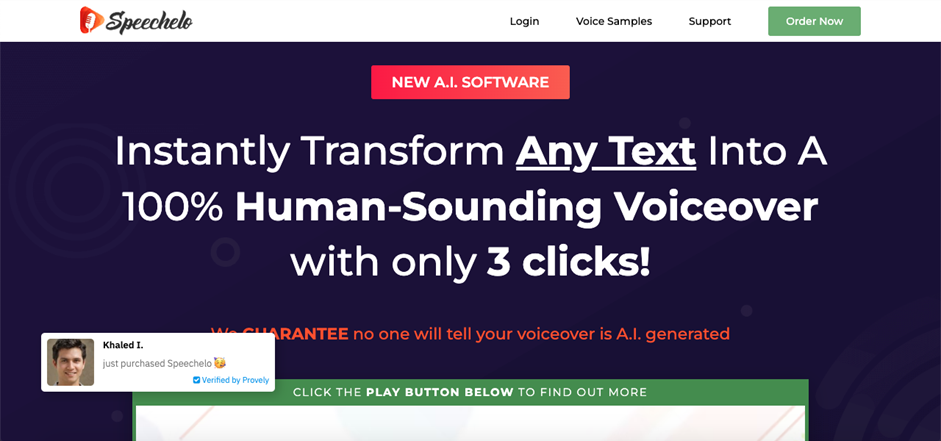The image showcases a website interface for SpeechLO. At the top left corner, there is a prominent red triangle icon resembling an old-fashioned radio microphone, indicating the brand's focus on voice technology. To the right of this icon are various navigational options in black text, including "Login," "Voice Samples," and "Support." A green rectangle labeled "Order Now" in white text is also prominently displayed for immediate access to purchasing options.

Below the navigation bar, a substantial navy blue banner stretches across the screen. Centrally positioned at the top of this banner is a clickable coral-colored rectangle with the text "New AI Software." Directly beneath this, in large, bolded white font, is the announcement: "Instantly transform any text into a 100% human-sounding voiceover with only three clicks," emphasizing the ease and authenticity of the software.

Further down, a testimonial quote from a user named Khalid is featured, affirming the software’s quality with the claim, "We guarantee no one will tell you your voiceover is AI generated." At the bottom of the banner, there is a call-to-action button inviting users to "find out more."